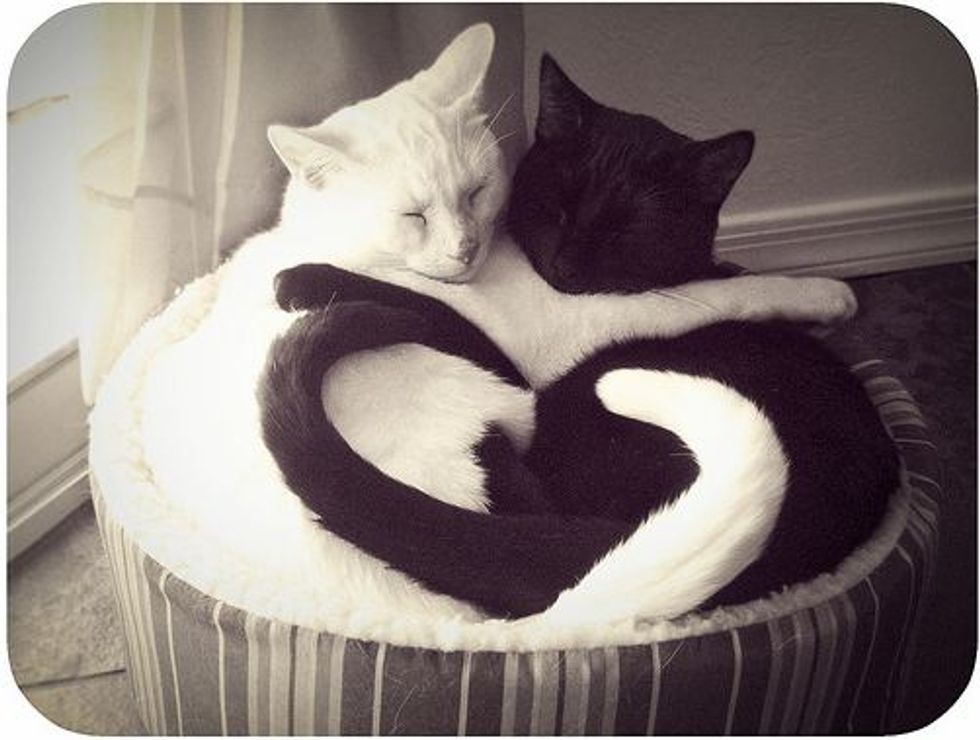In this detailed black-and-white photograph, two cats are nestled together in a striped pet bed material. The striped fabric of the bed has a vertical design, and inside the bed is soft, contrasting with its exterior. The cat on the left is white with its eyes closed, embracing the black cat on the right, whose eyes are also shut. Both cats have their arms wrapped around each other, creating a tender, intertwining posture. Their tails are curled gracefully in the foreground, forming a heart-like shape, though not quite fully connected. The cozy scene is situated next to a window with a white curtain, adding a touch of natural light to the intimate moment. In the background, a bit of carpet and a white wall are visible, completing the serene setting.